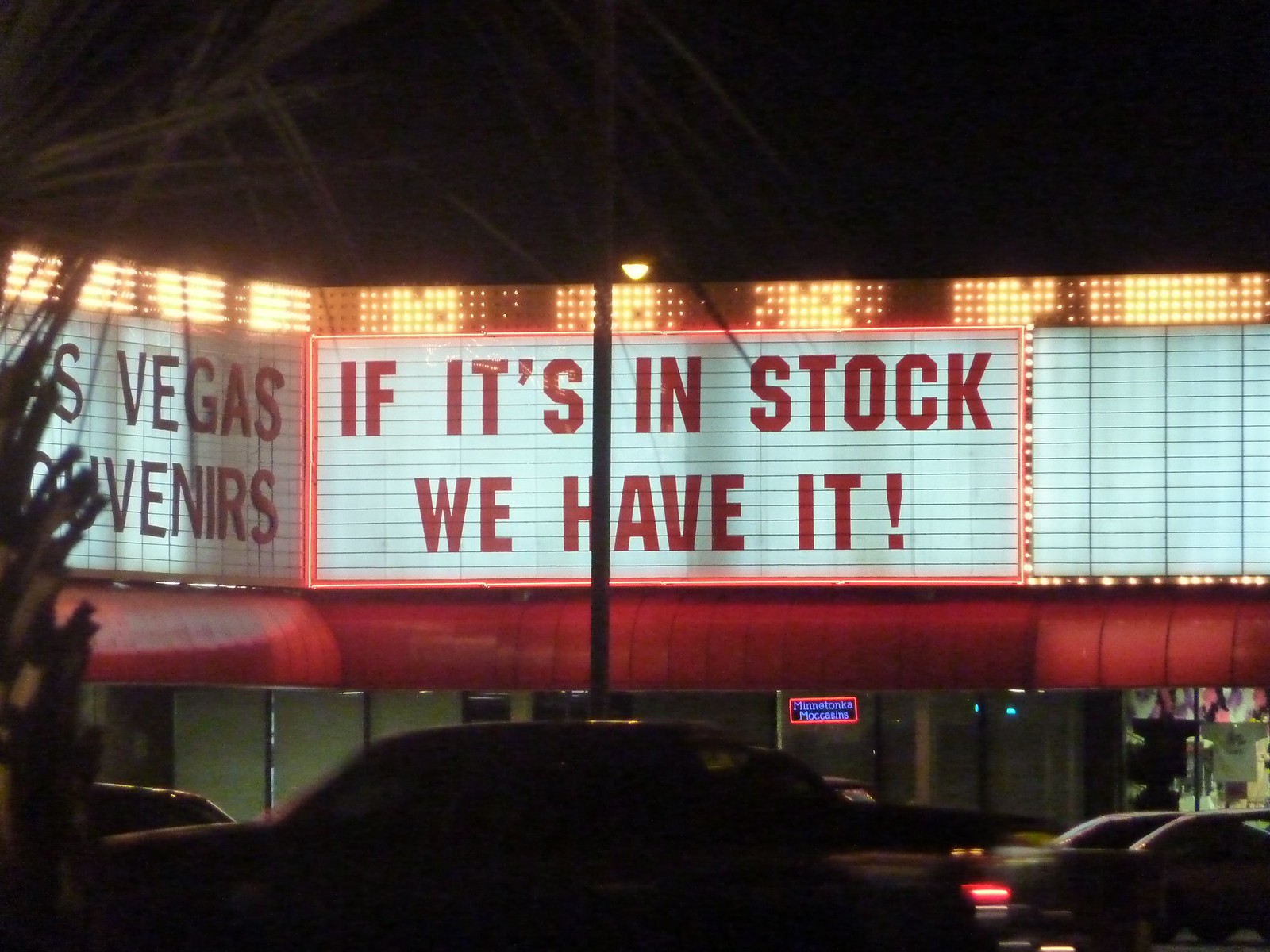The image captures a nighttime scene featuring a brightly lit building adorned with vivid signage and bustling with activity. At its center, a prominent sign styled like a theater marquee, with glittering lights and bold red lettering, declares, "If it's in stock, we have it!" Below the main sign, a red awning leads to an unclear storefront, suggesting a sense of mystery or curiosity about the establishment's offerings. To the left, an adjacent awning reads "Las Vegas Souvenirs," partially obscured by a tree but still discernible. Yellow lights illuminate the signs, adding to the vibrant atmosphere. Blurred cars passing by underscore the dynamic setting, reflecting the typical hustle and bustle of a lively Las Vegas night.